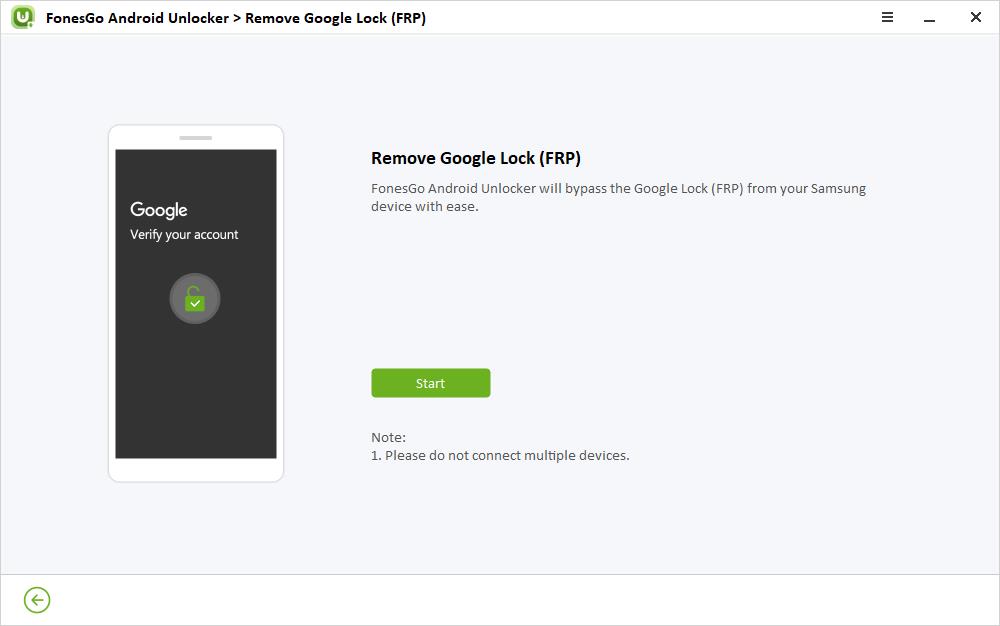The image features a user interface screenshot from an Android unlocking software. Central to the screen is a logo comprising a white "U" inside a green circle, distinctively different from its typical light green square background. The text prominently reads, "Phones Go, Android Unlocker: Remove Google Lock (FRP)," all in bold black lettering. Following this, three horizontal lines, a dash, and an "X" icon are displayed. 

Below a gray dividing line appears a depiction of a smartphone with a white body. The phone’s screen displays a message in white text on a black background that reads, "Google, Verify Your Account." Adjacent to this is a solid gray circle harboring a green padlock, which features a white checkmark in its center.

To the right of the phone image is a text block that states, "Remove Google Lock: Phones Unlocker will bypass the Google lock." Beneath this message is a green button with white text that says "Start." Further down, in gray text, is a cautionary note: "Note 1: Please do not connect multiple devices." Another gray dividing line follows, leading to a section of white space that includes a green circle with a green arrow inside.